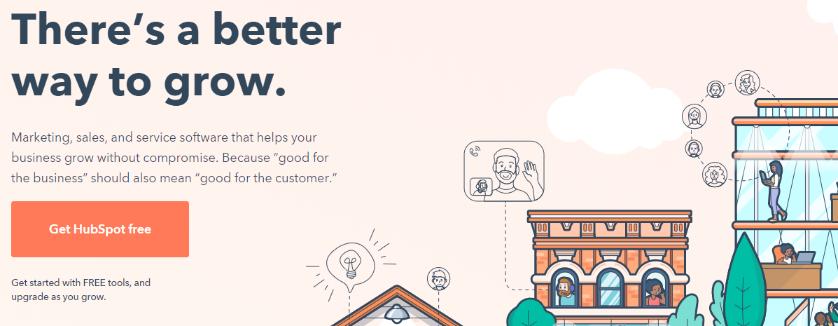This image features a well-structured and visually engaging promotional page for HubSpot. At the top left corner, the phrase "There's a Better Way to Grow" is prominently displayed in large, bold blue font. Directly beneath this headline, a succinct paragraph outlines the benefits of HubSpot's marketing, sales, and service software, stating, "A marketing, sales, and service software that helps your business grow without compromise. Because good for the business should also mean good for the customer."

An eye-catching orange, rectangular button is positioned below the text, containing the call-to-action "Get HubSpot Free" in white lettering. Further down in the bottom left corner, there’s additional guidance in smaller text that reads, "Get started with free tools and upgrade as you grow."

To the right of the text, there is an illustration set against a beige background featuring clouds in the sky and a series of three buildings that increase in height from left to right. The middle building, designed with numerous windows, depicts people engaged in various activities, including a person appearing to be on a conference call. The tallest building, characterized by extensive glass facades, includes an illustration of a ring of people's faces, suggesting collaboration, and individuals working in their offices. The buildings are complemented by trees planted in front, adding a touch of nature to the urban scene.